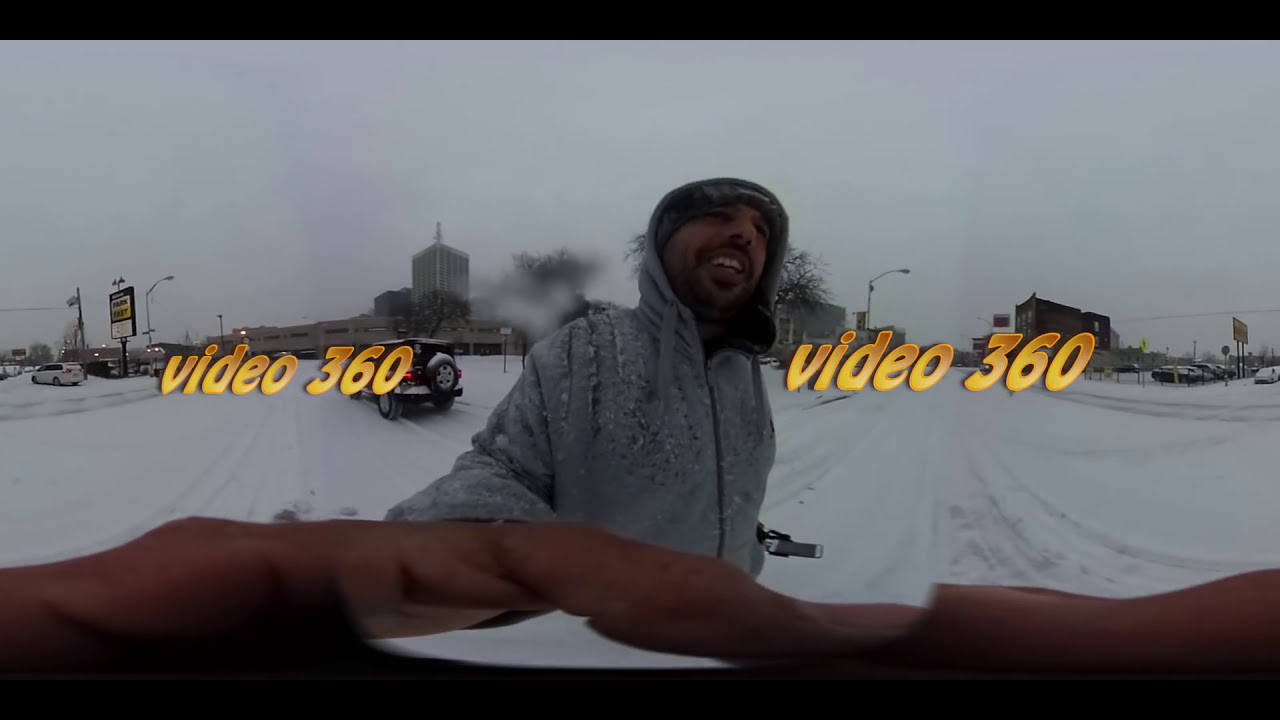The image shows a smiling young man wearing a gray coat and a dark knit cap, standing at the center of a snowy, overcast scene. He appears to be taking a selfie with a fisheye lens, causing a slight distortion of his hands reaching towards the camera at the bottom of the screen. Surrounding him is a clearly visible text in yellow reading "Video 360" on both the left and right sides of the image. The setting is an outdoor, snow-covered road with several vehicles, including a Jeep, in the background, along with buildings, street lamps, and signs. The sky above is a uniform gray, adding to the wintry atmosphere. The black border encompasses the image, giving it a framed appearance.